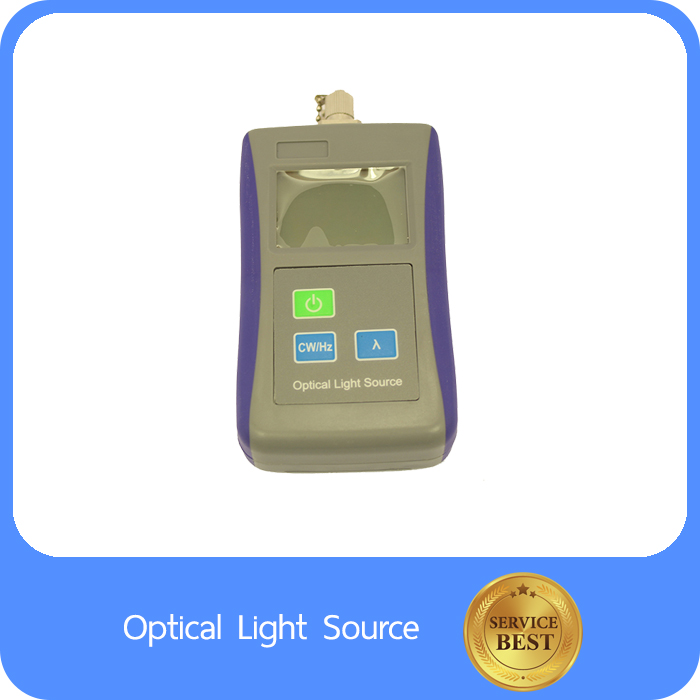This image depicts an advertisement for an optical light source device set against a predominantly white background with blue edging towards the bottom. The central focus is a gray, plastic device with purple sides and a clear glass section on top, covered by a plastic screen. The device features three buttons: a green power button located at the middle-left, a blue button labeled "CW/HC" below it, and to the right, another blue button marked with a symbol possibly representing ohms. Below these buttons, the text reads "optical light source." At the very bottom of the image, in a blue section with white text, the words "optical light source" are reiterated. Adjacent to this text is a gold circular emblem with the inscription "service best" in brown font, flanked by three stars on top and small feathers encircling the lower part of the disc.